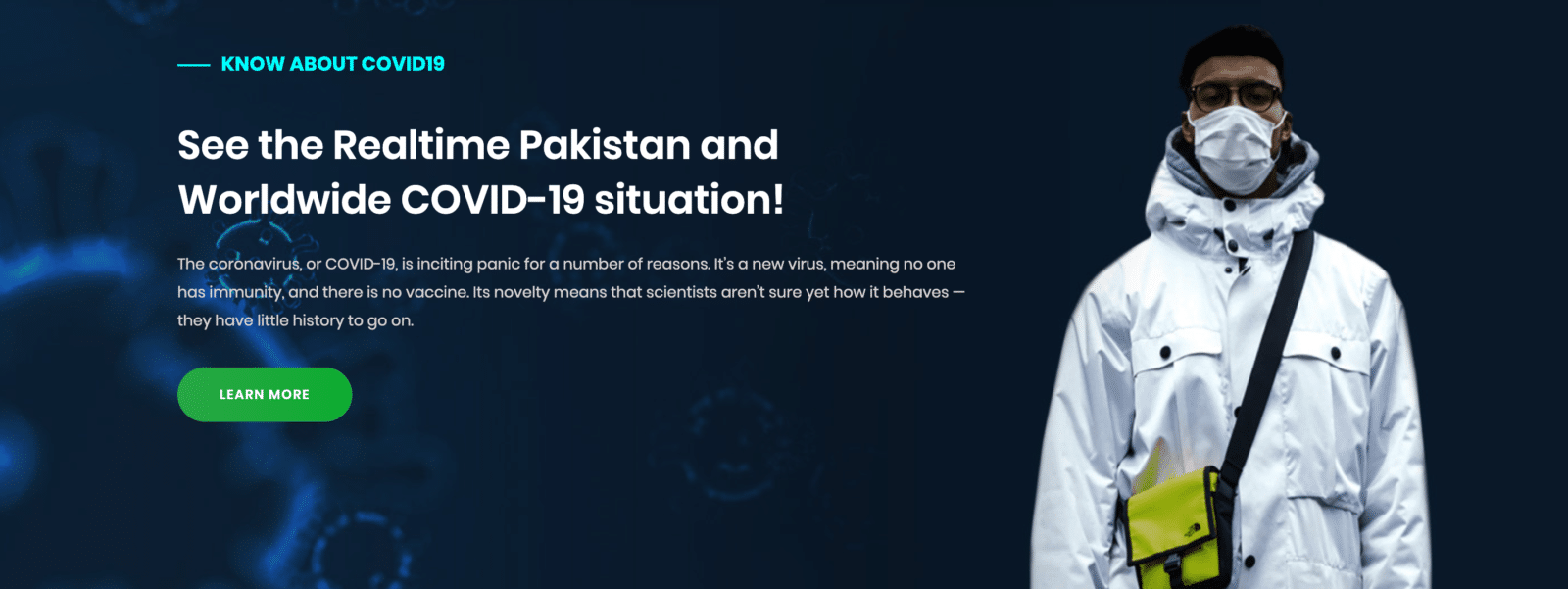A large rectangular screenshot showcasing part of a webpage detailing Pakistan's coronavirus response. The image features a dark blue background. On the right side, an Indian man dressed in medical attire — including a long white coat, a face mask, and a yellow shoulder bag — stands prominently. At the top left, bold light blue font text reads "Know about COVID-19." Just below, bold white font announces, "See the real-time Pakistan and worldwide COVID-19 situation," followed by a brief explanation in smaller white letters. Below this text, a green button on the left side displays "Learn more" in small white letters. The bottom left corner of the image is accented by a light blue, diagonally-oriented outline resembling cells.